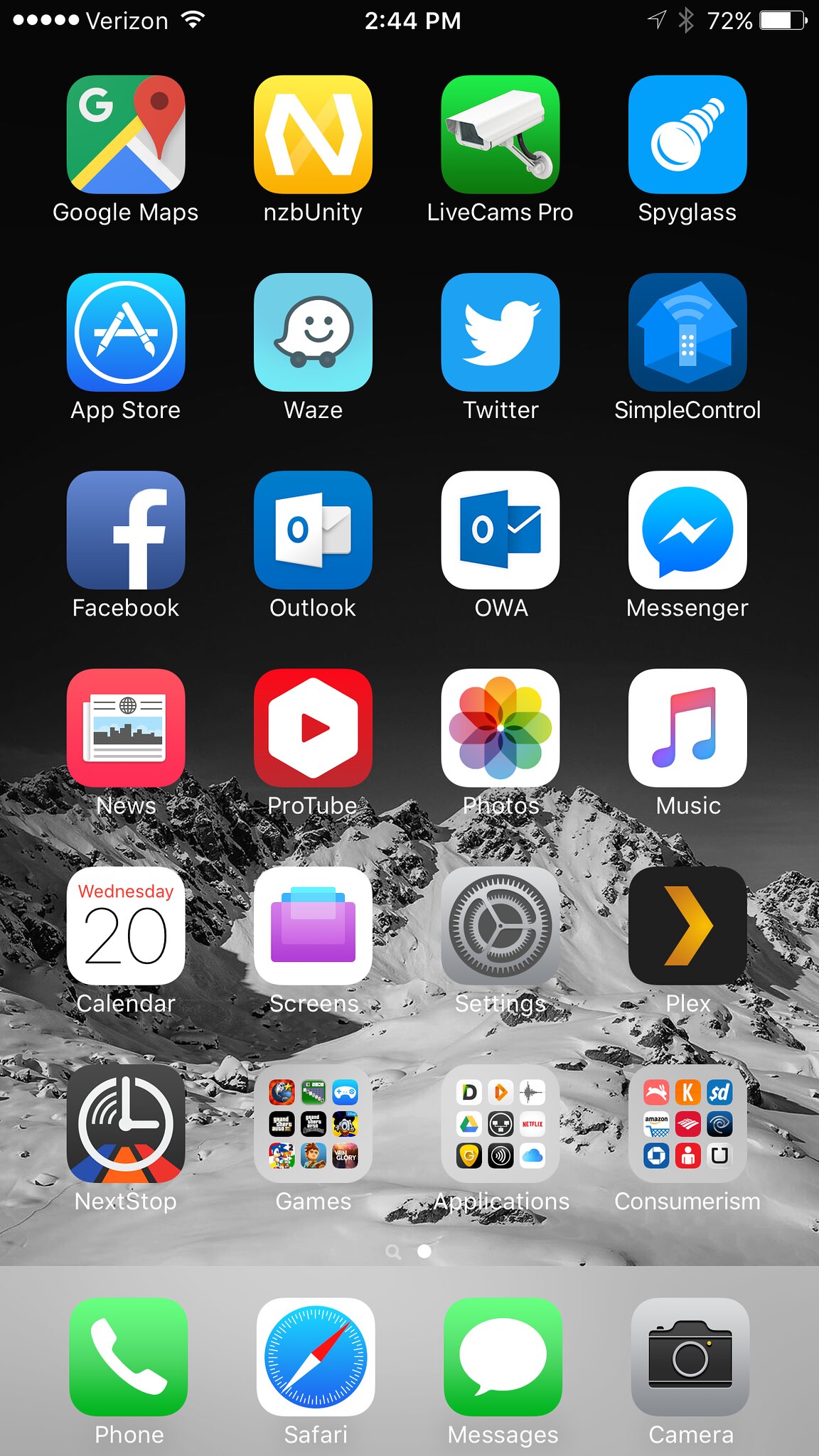This is a detailed description of a smartphone screen capture. The screenshot was taken at 2:44 PM, as indicated by the time displayed at the top center of the screen. To the top left, there are five white circles representing the phone’s signal strength, followed by the carrier name, Verizon. Over on the right side, a battery icon shows 72% remaining battery life.

The screen displays multiple app icons arranged in rows. On the top row, from left to right, there are the Google Maps app, the N2B Unity app, Live Cameras Pro, and Soy Glass. The second row features a blue box icon (the specific app is not named), the App Store app, Waze, Twitter, and Simple Control. 

In the third row, the apps include Facebook, Outlook, OWA, and Messenger. The fourth row contains the Notes app, ProTube, Photos, and Music. The fifth row displays the Calendar app, which shows "Wednesday the 20th," a white box with a blue folder labeled "Screens," the Settings app, and the Plex app. 

The bottom row includes folders labeled Games, Applications, and Consumerism. Along the bottom dock area, there are four frequently used apps: Phone, Safari, Messages, and Camera, from left to right.